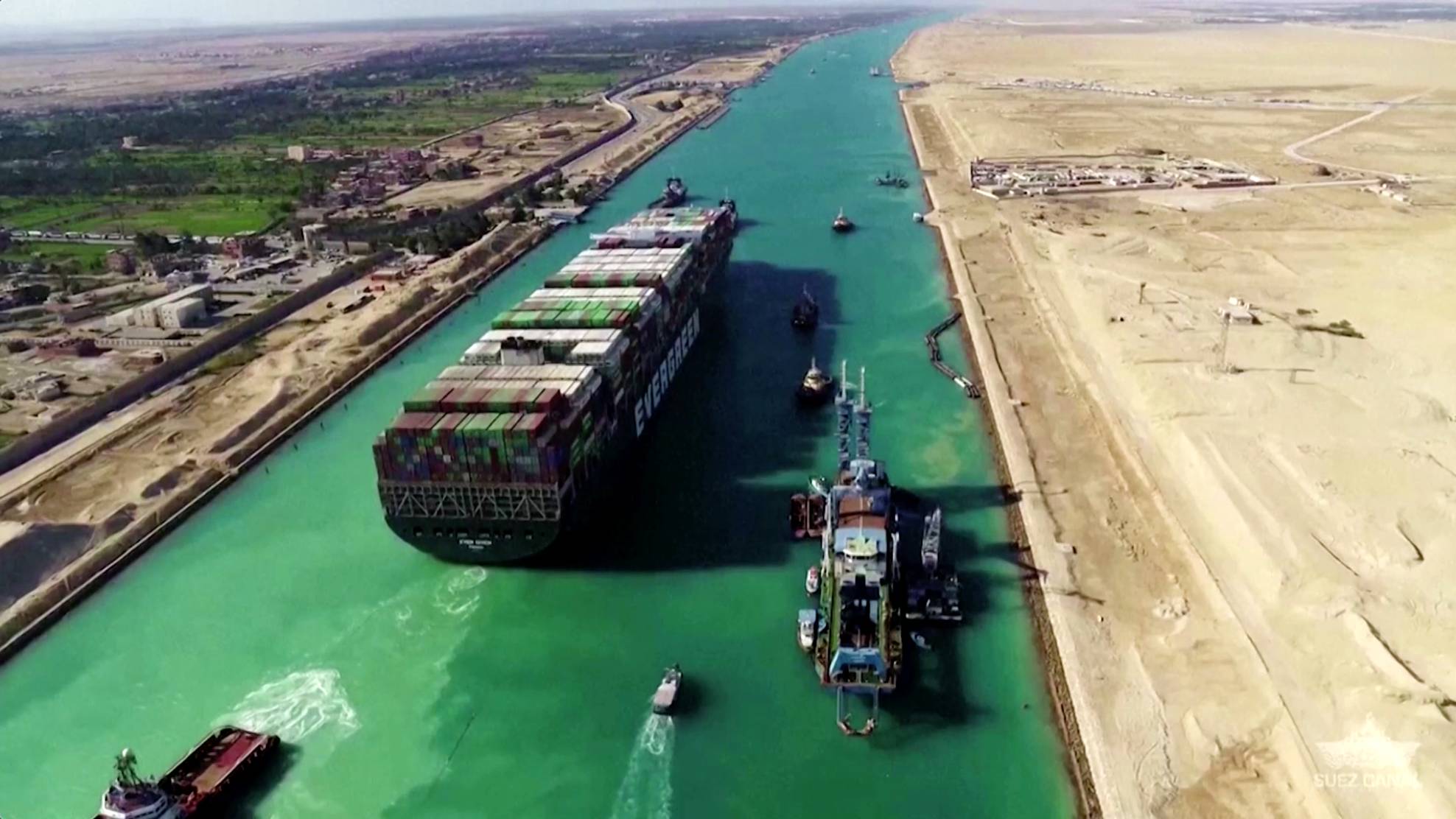This aerial image taken in daylight captures a busy canal, resembling a shipping or operational port. The expansive waterway, possibly a canal or sea channel, is flanked by contrasting landscapes: a barren, desert-like area with unidentifiable structures on the right, and a verdant strip with green trees and several rounded tanks, possibly for storage, on the left. Dominating the canal is a massive barge named "Evergreen," heavily loaded with shipping containers stacked two or three high, accompanied by smaller boats and tugboats aiding its navigation through the narrow passage. In the distance, there are patches of grassy fields and dirt areas, alongside roads with vehicles and scattered buildings, suggesting an operational zone with office structures and port facilities. Additionally, another smaller ship trails behind the large barge, emphasizing the active maritime traffic in the canal.